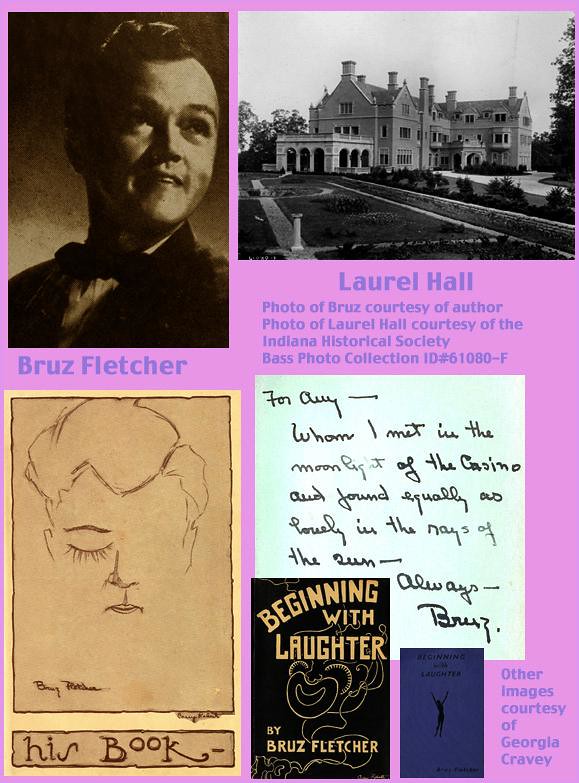This image is a detailed collage on a light lilac background, arranged in a portrait layout with a variety of visual and textual elements. In the upper left corner is an old sepia-toned headshot of a man named Bruce Fletcher, who appears to be of Caucasian descent, wearing a suit with a bow tie and looking slightly to the right. Beneath this photograph, there is a partially drawn caricature that mirrors Bruce's face, showing only one eye, part of the nose, and the mouth on an old piece of parchment. In between these images, it reads "Bruce Fletcher." 

In the upper right corner, there is a black-and-white photograph of a grand mansion labeled "Laurel Hall," with the caption noting that the photo is courtesy of the Indiana Historical Society, collection ID number 61080-F. Below this, a handwritten note reads, "For Amy, whom I met in the moonlight of the casino and found equally as lovely as the rays of the sun. Always, Bruce," indicating a personal message from Bruce Fletcher.

At the bottom of the collage, there is a dark purple rectangle with the title "Beginning with Laughter" in orange writing, which appears to be the cover of a book by Bruce Fletcher. Adjacent to this, another text block credits other images to "Georgia Crabby." The combination of photographs, drawings, and handwritten notes, along with detailed labels, provides a historical and personal narrative centered around Bruce Fletcher and his work.